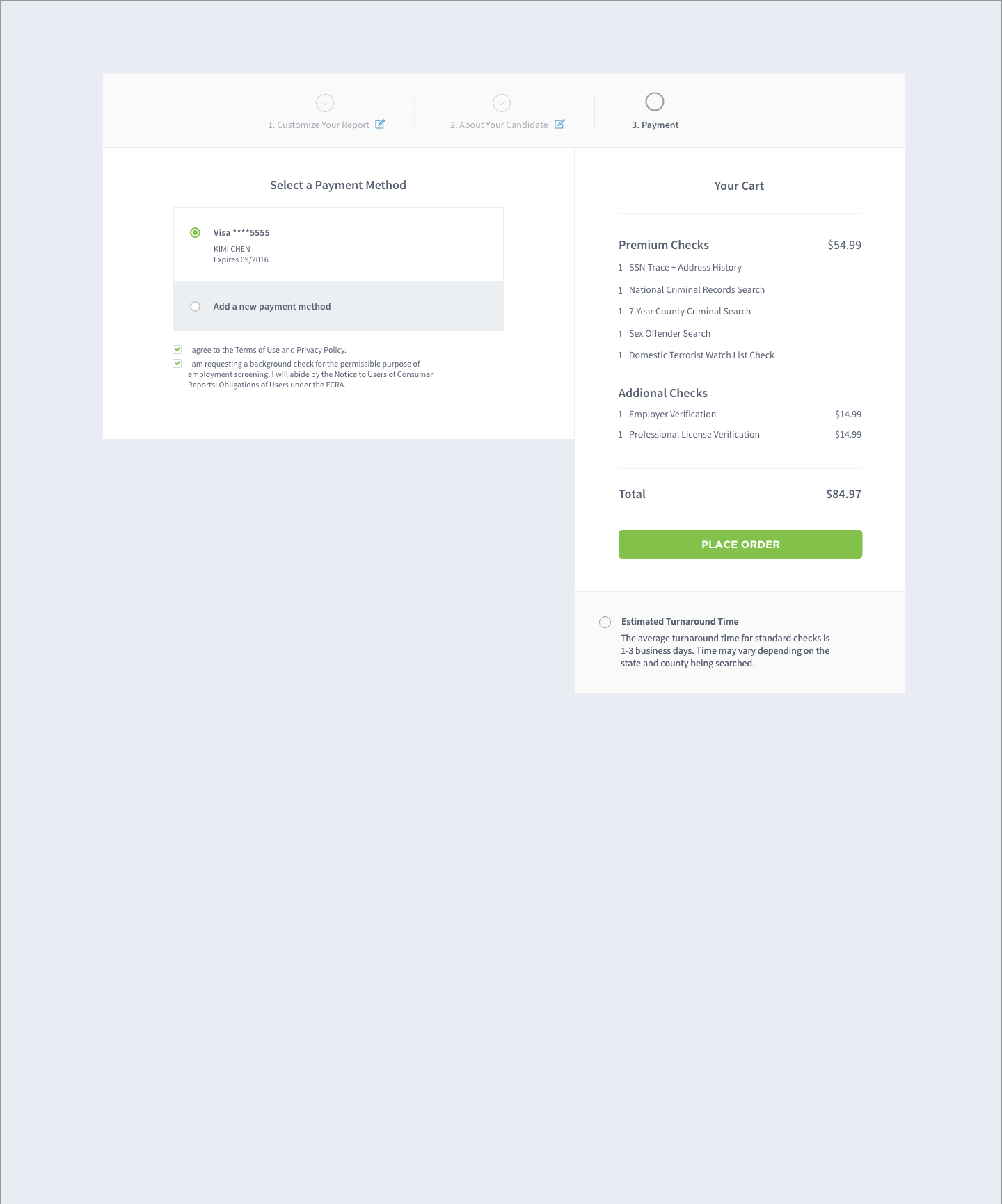A screenshot of an online payment page displaying a step-by-step guide for purchasing a candidate report. At the top, the text reads:

1. Customize your report.
2. Buy your candidate.
3. Payment.

Highlighted in green is a prompt: "Select Payment Method." Below, a green dot indicates a selected Visa card ending in 5555, belonging to Qimu Tran, with an expiration date of 09/02/16. Additional text offers the option to "Add a New Payment Method," and an agreement checkbox states: "I agree to the Terms of Use and Privacy Policy. I request a background check for the purpose of employment screening. I acknowledge the notice to use a consumer report. Submissions are used under the FCRA."

Details of the chosen report include:
- Premium Tax: $54.99
- 1 SSN Trace plus Address History
- 1 National Criminal Records Search
- 1 7-Year County Criminal Search
- 1 Sex Offender Search
- 1 Domestic Terrorist Watch List Check

Additional checks include:
- 1 Employer Verification: $14.99
- 1 Professional License Verification: $14.99

The total cost is displayed in gray text: $84.97. At the bottom, a green button labeled "Place Order" is visible. Gray text also shows the estimated turnaround time: "The average turnaround time for standard checks is 1 to 3 business days. Time may vary depending on the state and county being searched."